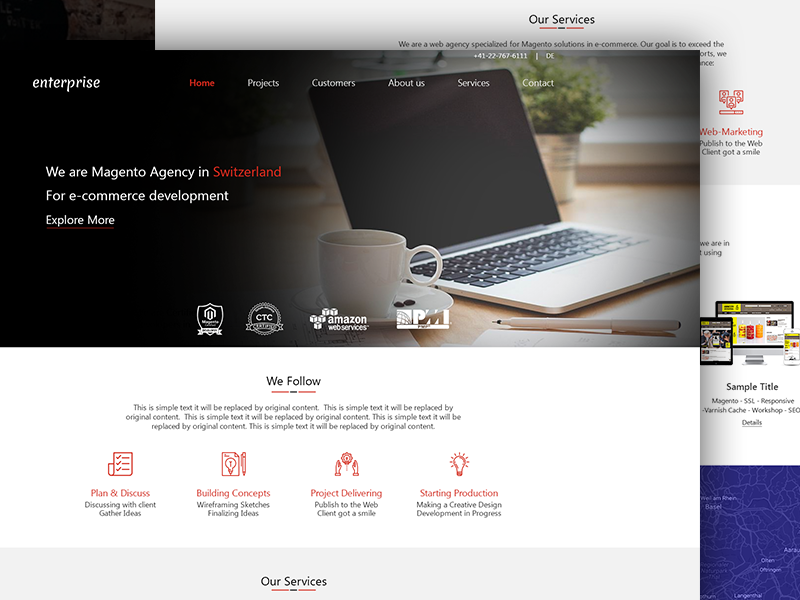In the upper left corner of the image, the word "Enterprise" is displayed in white, followed by a horizontal list of navigation options: "Home," "Projects," "Customers," "About Us," and "Services." The "Home" link is highlighted in red, while the others remain white. Below this, there's text declaring, "We are a Montego agency in Switzerland for e-commerce development. Explore more." The image itself is a photograph featuring a laptop and a cup of coffee, with the writing placed on a darkened left side that fades to black. 

Underneath this text, there are several icons: one is illegible, one reads "CTC," another is labeled "Amazon Web Services," and the fourth says "PM." Further down, on a white background, the phrase "We follow. This is a simple test, it will be replaced by original content. This is a simple test," repeats multiple times, indicating this section is a placeholder for future content. 

At the bottom of this template, there are four red icons accompanied by headers and black descriptive text below each: "Plans and Discuss," "Build Concepts," "Project Delivering," and "Start Production." Below this section, a header reads "Our Services," which is also partly visible on the right side of the image but obscured by overlapping elements.